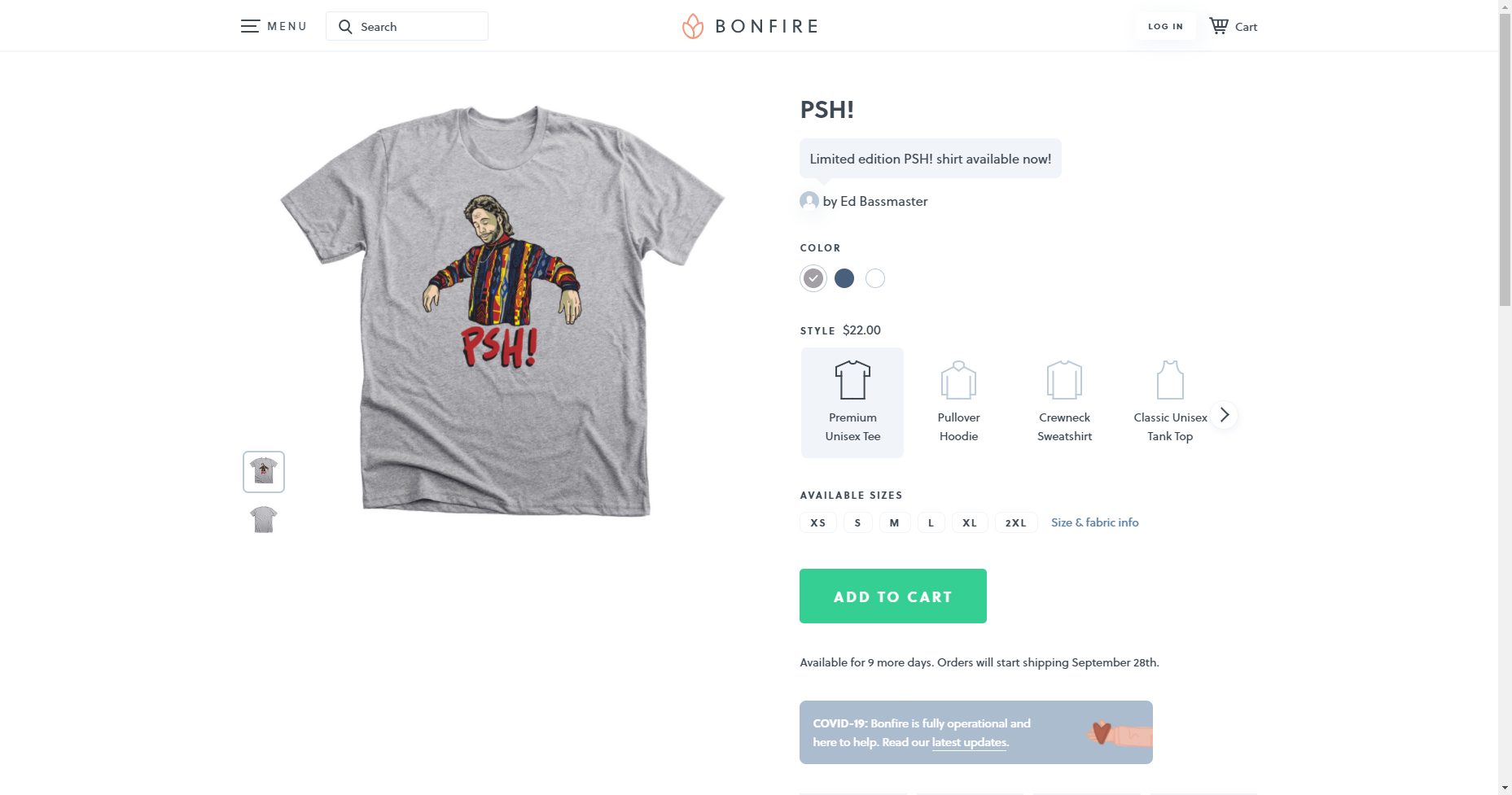This detailed image captures the website interface of Bonfire. The top left features a menu bar with several icons and a search bar. The logo, which resembles a gold leaf with the company name "Bonfire" in white capital letters, is prominently displayed.

To the right of the logo, there are buttons for logging in and accessing the shopping cart. 

The highlighted product is a gray t-shirt. This t-shirt is showcased through two images: a smaller, square image at the top (presumably the front view) and a larger image below (likely the back view). The front of the shirt is adorned with the word "Psh" in red letters, complete with an exclamation point. Above this text, there's an illustration of a man dressed in hippie-style long-sleeve attire with long hair.

To the right of the images, a description box reads: "Psh! Limited Edition. Available Now." Following this, there is information about the designer, Ed Bassmaster, and the color options available: gray, blue, and white.

The product offers a range of types, including a unisex top, hoodie, sweatshirt, and tank top, with sizes ranging from extra small (XS) to extra-extra-extra-large (XXXL). The "Add to Cart" button is prominently displayed in a green color, inviting users to make their purchase.